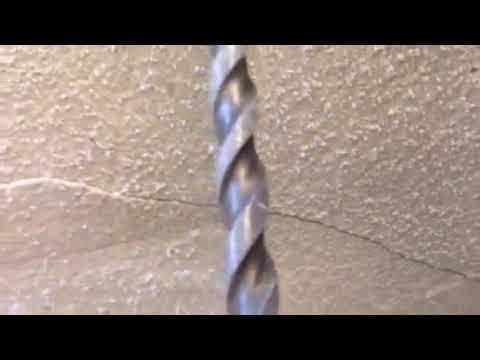This image, a horizontally-aligned, smaller rectangular picture, features pronounced black borders at the top and bottom, reminiscent of letterbox movie bars. The central section showcases a textured backdrop resembling a light gray, cracked masonry or cement wall. The crack originates from the lower right, curving up to the center before extending towards the left side, resembling a fault line. Dominating the central vertical axis of the image is a silver, cylindrical bit, seemingly designed for drilling into masonry. This tool has a smooth, helically twisted surface with raised sections in between. Notably, the bit appears stationary, and its extremities are hidden by the borders, presenting a close-up view of its midsection. The scene evokes a sense of active drilling, despite the absence of the drill itself, leaving viewers to infer ongoing action from the prominent spiral bit and the visible crack in the textured wall.